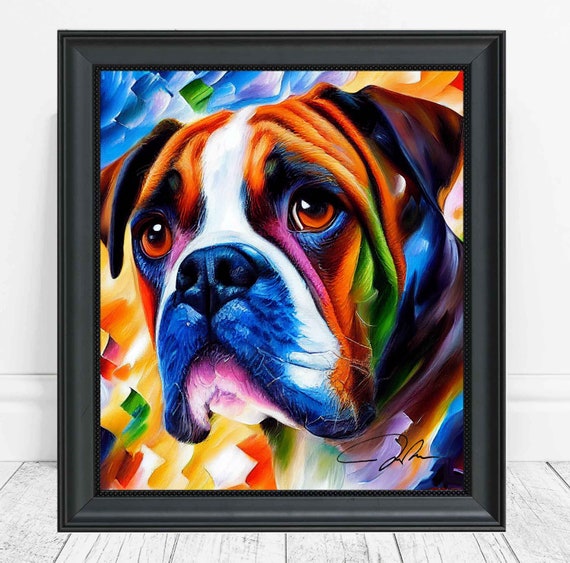The image depicts an impressive and vividly colored painting of a dog, likely a boxer, displayed in a black wooden frame. The background setting includes a pristine white wall with white wooden flooring, giving a stark contrast to the colorful artwork. The dog’s face is the focal point, characterized by droopy jowls and a somber expression, highlighted by its light brown eyes that appear to be looking off into the distance. The dog features a mix of colors, including a prominent white stripe between its eyes, with shades of blue on the cheeks, and green spots on its right cheek, under its eyes, and below its lower jaw. The nose is black, and the mouth is closed in a typical frown, giving it a realistic appearance enhanced by detailed fur texture, particularly around the nose. The vibrant background employs short brush strokes with hues of yellow, red, green, purple, and blue, creating a dynamic and eye-catching contrast. The painting's signature is visible in the bottom right corner, suggesting it is a professionally done piece. The overall composition suggests that the piece could be a showcase item for an online shop, emphasizing the high quality and artistic craftsmanship.